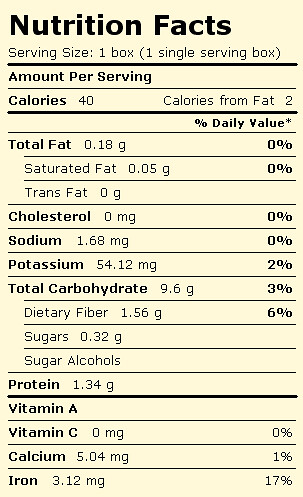The image portrays a standard U.S. nutrition facts label with a beige background and black text. It indicates that the serving size is one single-serving box. The nutritional information is as follows: 40 calories per serving, with 2 calories from fat. The total fat content is 0.18 grams (0% daily value), including 0.05 grams of saturated fat (0%), and 0 grams of trans fat. Cholesterol content is 0 milligrams (0%). The label lists 1.68 milligrams of sodium (0%) and 54.12 milligrams of potassium (2%). Total carbohydrates are 9.6 grams (3%), which includes 1.56 grams of dietary fiber (6%) and 0.32 grams of sugars. Protein content is 1.34 grams. Vitamins A and C are absent, while calcium is present at 5.04 milligrams (1%) and iron at 3.12 milligrams (17%). Overall, the product appears to offer minimal nutritional value aside from its iron content.